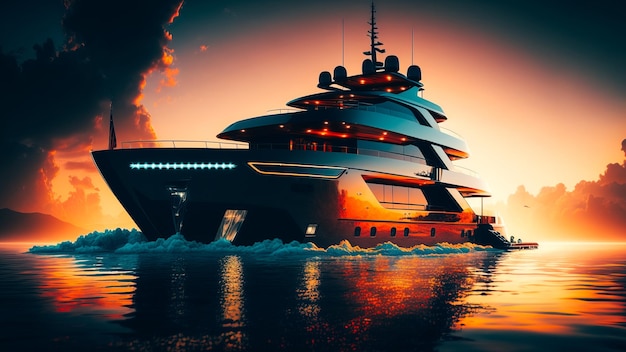The image depicts a computer-generated rendering of a luxurious yacht, resembling a millionaire's vessel, prominently positioned in the center. The yacht features three distinct decks and seems to be navigating slightly leftward, with its bow on the left and stern on the right. Surrounding the yacht is an intense, foamy white water, suggesting motion, although the foam's unusual distribution implies an AI-generated origin.

The scene is bathed in a warm, orangish light, indicating either sunrise or sunset. This illumination enhances the dramatic silhouette of the yacht against the sky. At the base level, a platform sits at the waterline, leading up to an expansive open bow and an enclosed section towards the vessel's middle and rear. Above, the second deck likely houses the captain’s area, featuring a small, open balcony, while the third deck could serve as storage or an additional navigational space, marked by various instruments and a prominent antenna.

In the surrounding landscape, dark puffy clouds loom on the horizon, adding depth and drama to the sky. To the left, distant land and to the right, trees create a faint backdrop against the illuminated water. The water surface reflects the yacht, with the light suggesting the sun being positioned directly behind the vessel, enhancing the scene's serene yet dynamic quality.